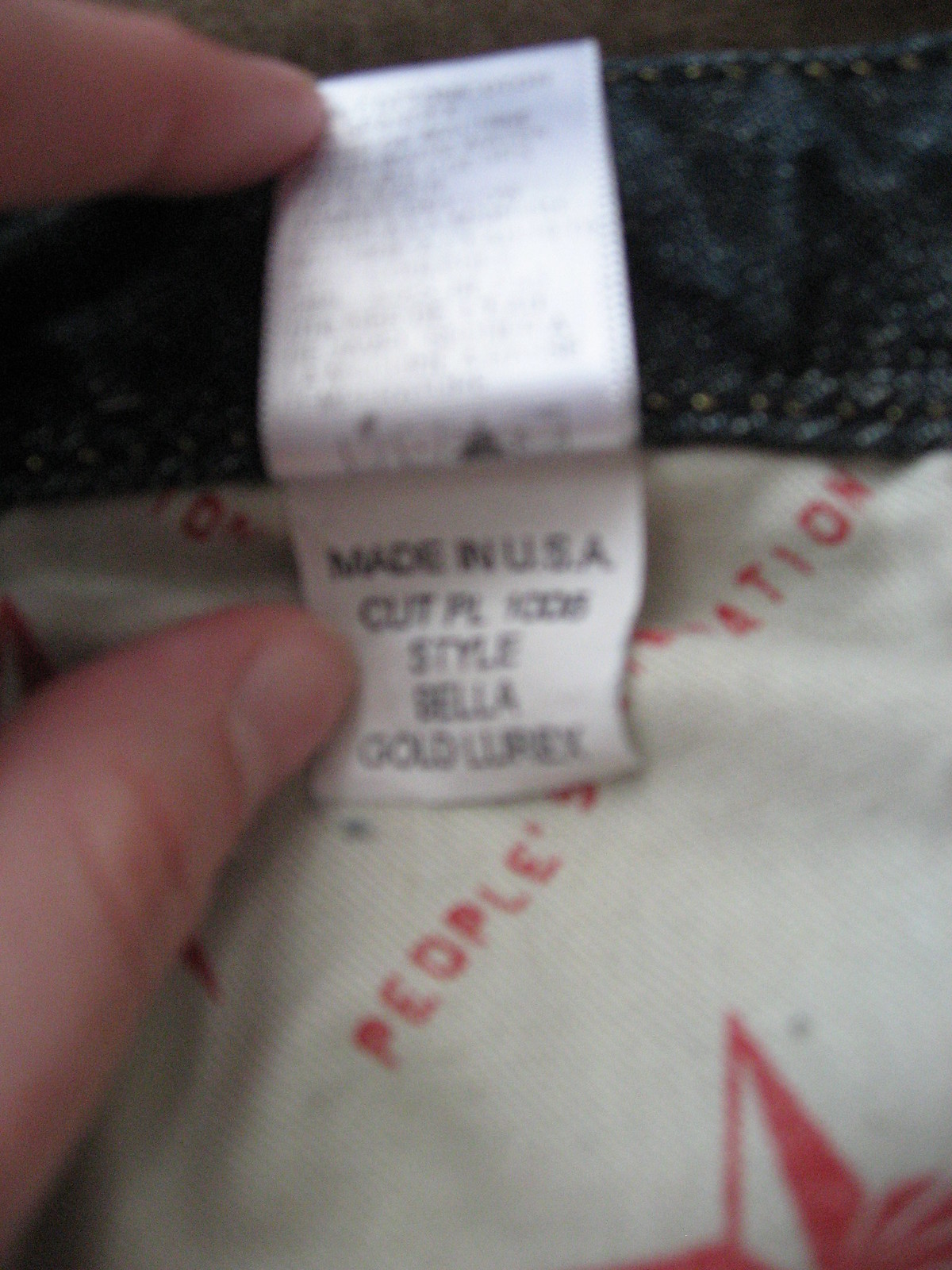In this slightly blurry image, a pair of blue jeans is being displayed with a focus on the interior tag. A Caucasian individual’s thumb and index finger are holding the white tag open. The tag, which has black text, reads "Made in USA" and includes mentions of "cut" and "style" with the word "Bella" noted, although the rest is too unclear to decipher. Additionally, the inner pocket lining of the jeans features red lettering that appears to spell out "People's Station," accompanied by a red star beneath the text, all set against a white fabric. The jeans are characterized by yellow stitching, and the background of the image is dark. The tag has more information on its reverse side, but it is not visible in this shot.